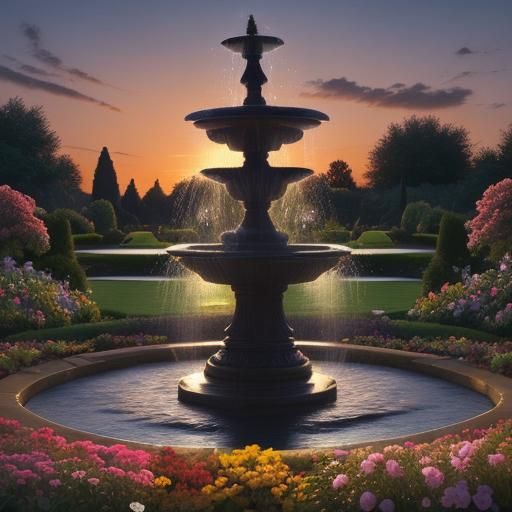The image, potentially a photograph or an artistic drawing, depicts a serene outdoor scene during sunset. In the foreground, a multi-tiered fountain with four bowls cascades water from top to bottom, each level progressively larger, finally emptying into a surrounding pond. Enclosing the pond’s concrete edge are vibrant flower beds featuring a mix of pink and yellow blossoms. Immediately behind the pond, there's a lush patch of green lawn leading to a distant tree line, which includes various types of trees, such as pines, and meticulously shaped hedges. The sky above, painted with a gradient of colors from orange and yellow near the horizon to deeper purple and blue hues higher up, is punctuated by the glow of the setting sun and two clouds flanking the fountain. This detailed and colorful scene captures the tranquil beauty of nature illuminated by the soft, ambient light of dusk.